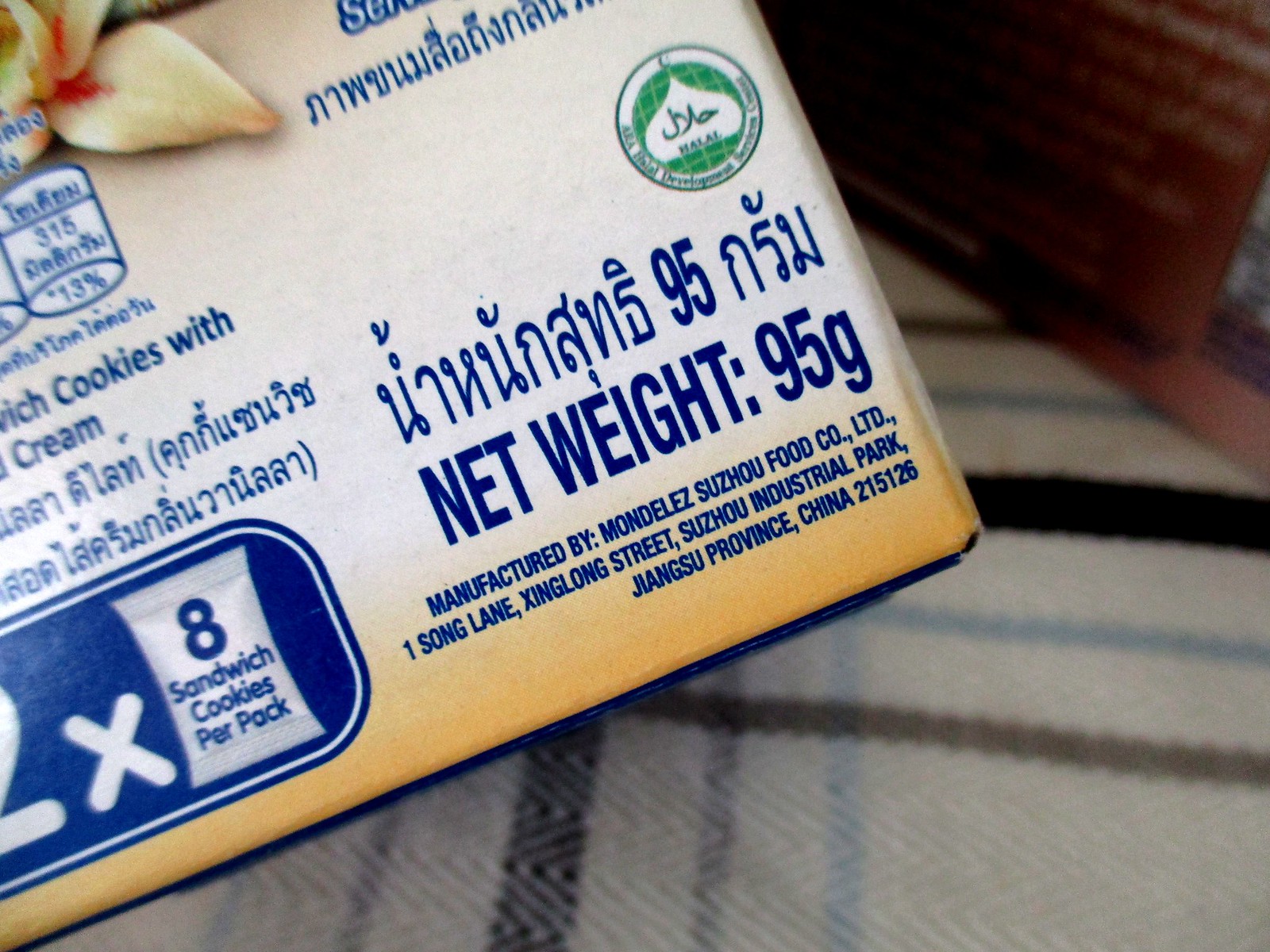This detailed color photograph captures a corner of a sandwich cookie packaging box. Predominantly white and yellow, the box features a variety of text and icons. Centered and diagonally across the image is the text "net weight 95g," and below it in blue reads, "manufactured by Mondelez Suzhou Food Co. Ltd., Wanzhong Lane, Xinglong Street, Suzhou Industrial Park, Jiangsu Province, China 215-126." In the bottom left, there's an oval rectangle housing an "X" alongside an illustration of a packet that states "2x 8 sandwich cookies per pack." Notably, the image includes East Asian text characterized by curves, circles, and arches, with a badge that says "hello" on the upper portion. On the right side, a partial view of a vanilla flower icon and various nutrition value symbols are visible. The upper right corner features additional East Asian characters, while the bottom right contains a green logo without English text. Surrounding the box, there's a blurred blanket in the right corner and another food product in the background, adding depth to the composition.